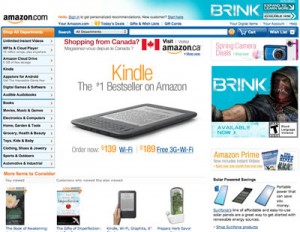This image depicts a section of a webpage from Amazon.com, showcasing a Kindle e-reader. The image is relatively small and the text is somewhat blurry and tiny, making it challenging to read. At the center of the page, there is a black Kindle device displayed on a white surface, showing text on its white screen. Above the Kindle, the word "Kindle" is prominently displayed in large orange text. Below this, in black text, it states "The Number One Bestseller on Amazon." Further down, the text reads "Order Now" in black, accompanied by the price "$139" in orange text for the Wi-Fi model. To the right, it lists "$189" in orange text for the Free 3G Wi-Fi model. Surrounding this main focus, there are various suggestions for other products displayed to the right and below the Kindle advertisement.